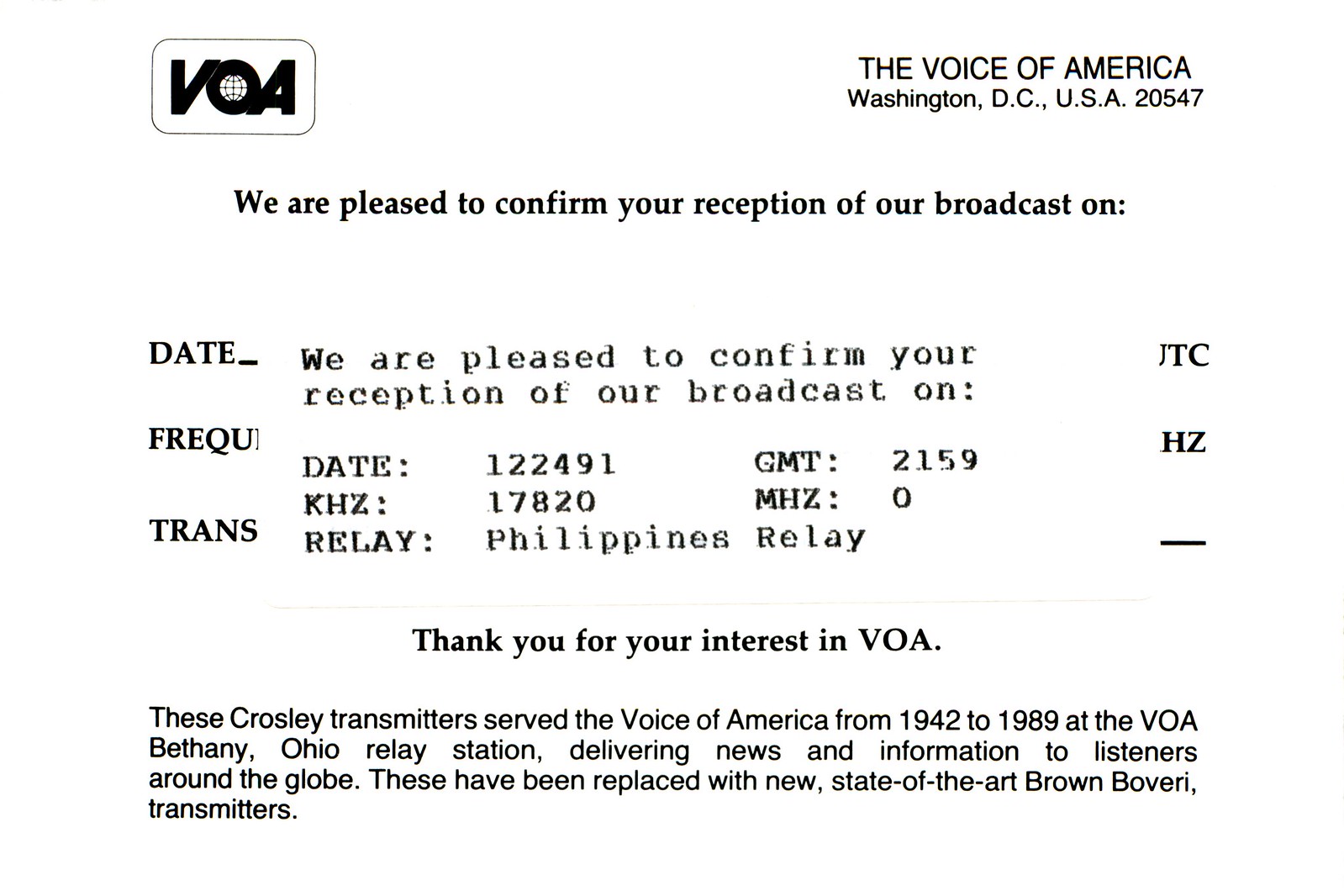The image depicts a scanned black-and-white document on a white background with plain black text. In the top left corner, there is a black logo with the letters "VOA." On the top right, it reads "The Voice of America, Washington, D.C., USA, 20547." Centered at the top, the text states, "We are pleased to confirm your reception of our broadcast on," followed by space for the date. Below this, specific broadcast information is listed: "Date 122491, GMT 2159, KHZ 17820, MHZ 0, Trans Relay, Philippines Relay." At the bottom of the page, in dark letters, it says, "Thank you for your interest in VOA." Further down, it details, "These Crosley transmitters served The Voice of America from 1942 to 1989 at the VOA Bethany, Ohio Relay Station, delivering news and information to listeners around the globe. These have been replaced with new state-of-the-art Brown-Boveri transmitters."